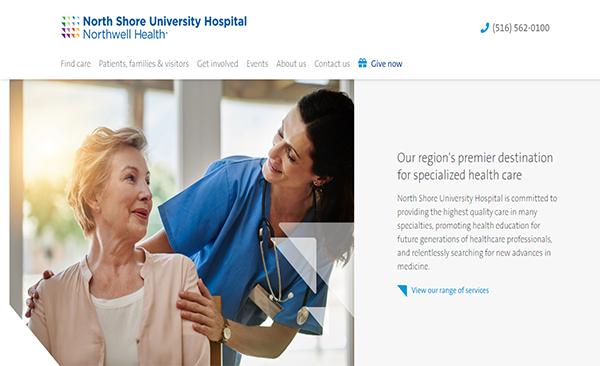This image is a screenshot from the North Shore University Hospital website. At the top of the page, there's a series of small, multicolored triangles in green, blue, orange, red, purple, and yellow. Adjacent to these triangles, there is blue text that reads "North Shore University Hospital" in a bold, prominent font, resembling Boulder type. Beneath the hospital's name, there is lighter, fainter blue text that says "Northwell Health."

Further down, the website displays a telephone icon next to the hospital's contact number, (516) 562-0100. Below the contact information, there are navigation links for various sections of the website, including "Find Care," "Patients, Families, and Visitors," "Get Involved," "Events," "About Us," "Contact Us," and "Give Now," with the "Give Now" link highlighted in blue text.

The central part of the screenshot includes an image of a caretaker attending to a seated patient. Next to this image, within a small gray square, is a message describing North Shore University Hospital's dedication to specialized health care. The text states: "Our region's premier destination for specialized health care. North Shore University Hospital is committed to providing the highest quality care in many specialties, promoting health education for future generations of health care professionals, and relentlessly searching for new advances in medicine." 

Lastly, there is a blue triangle with white text that calls to action: "View Our Range of Services."